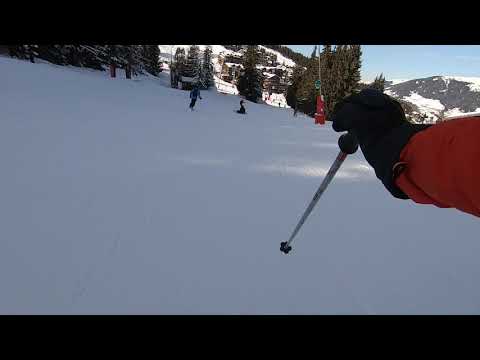This photograph, likely taken by someone skiing, captures a vivid winter mountain scene. Dominating the lower half of the wide, rectangular image is a blanket of crisp, white snow, with some areas shaded gray by the shadows. In the foreground, an arm clad in a red coat and black gloves extends from the right side, gripping a ski pole, suggesting the perspective of an active skier. The mid-ground is populated with other skiers, some appearing to navigate the slopes while one person seems to be on the ground. To the left, diagonally descending tall green pine trees, dusted with snow, add depth and contrast to the scene. On the far right, a blue sky merges with a majestic, gray mountain. A small red structure on the right side hints at a ski station. The entire image is subtly bordered by thin black strips at the top and bottom, framing this lively snapshot of a sunny day on the slopes.